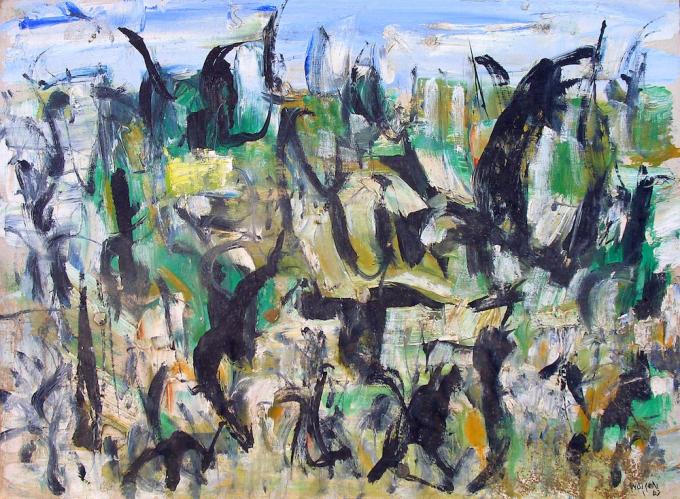This abstract painting features a blurred, almost impressionistic background with green lines that suggest the slender trunks of trees. The scene is energetically punctuated by a chaotic web of black brushstrokes that crisscross in various directions, resembling a frenetic dance of abstract figures in motion. These figures, reminiscent of rudimentary human forms, evoke a sense of activity and energy, appearing to wave their arms or perform handstands. The background is a patchwork of color with a yellowish hue that might represent arid grasslands or desert terrain, transitioning into streaks of blue sky at the top. Towards the bottom of the painting, there are warmer shades of orange and yellow. There's a colorful interplay of greens and yellows towards the center and bottom, while blues dominate the left and upper areas. Amidst this vivid scene, there’s a subtle attempt at text in the center of the painting, with discernible letters like "Y," "I," and "R," though they are partially obscured by the surrounding brushstrokes.